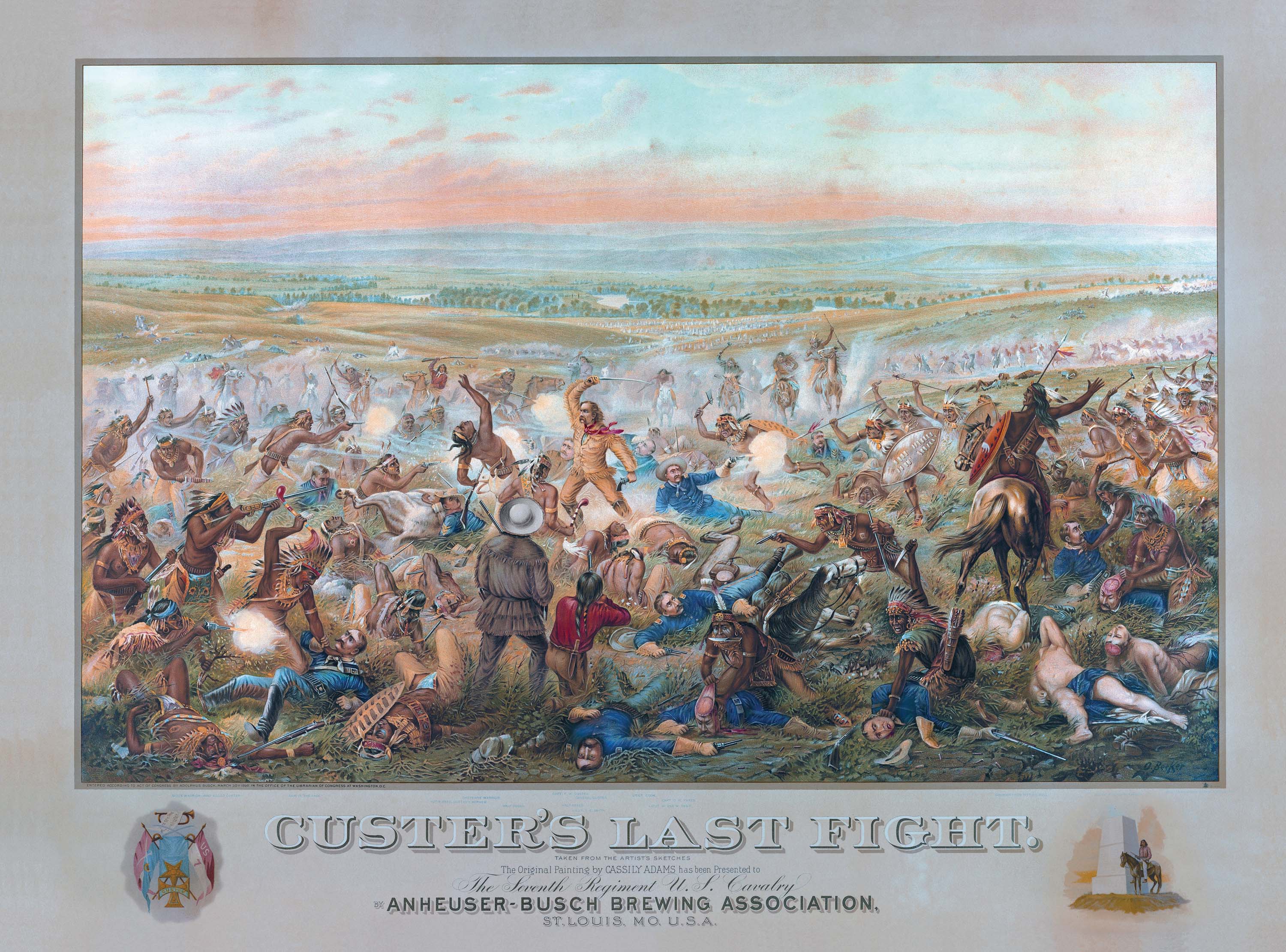This richly detailed poster features a central painting titled "Custer's Last Fight," bordered by a prominent silver frame. The painting vividly portrays the chaotic and brutal battle between Custer's cavalry, clad in blue uniforms, and the opposing Native American forces, many of whom are shown bare-chested and valiantly fighting on horseback. Central to the scene is Custer himself, distinguishable by his raised bayonet and red scarf, valiantly fighting amidst the turmoil. The battlefield is littered with fallen soldiers and Native Americans, highlighted by contrasting splashes of brown, blue, and red.

Beneath the central image, the text "Custer's Last Fight" is prominently displayed in white, outlined in black, with additional inscriptions that read "Anheuser-Busch Brewing Association, St. Louis, Missouri, USA". On the right side of the border is a smaller image of a Native American warrior riding a horse, positioned near three white brick blocks. On the left side, a crest is displayed above red and blue flags. In the distance, more Native American warriors can be seen charging through a pink and blue sky. The dramatic backdrop of green hills and trees further intensifies the grimness of the scene.